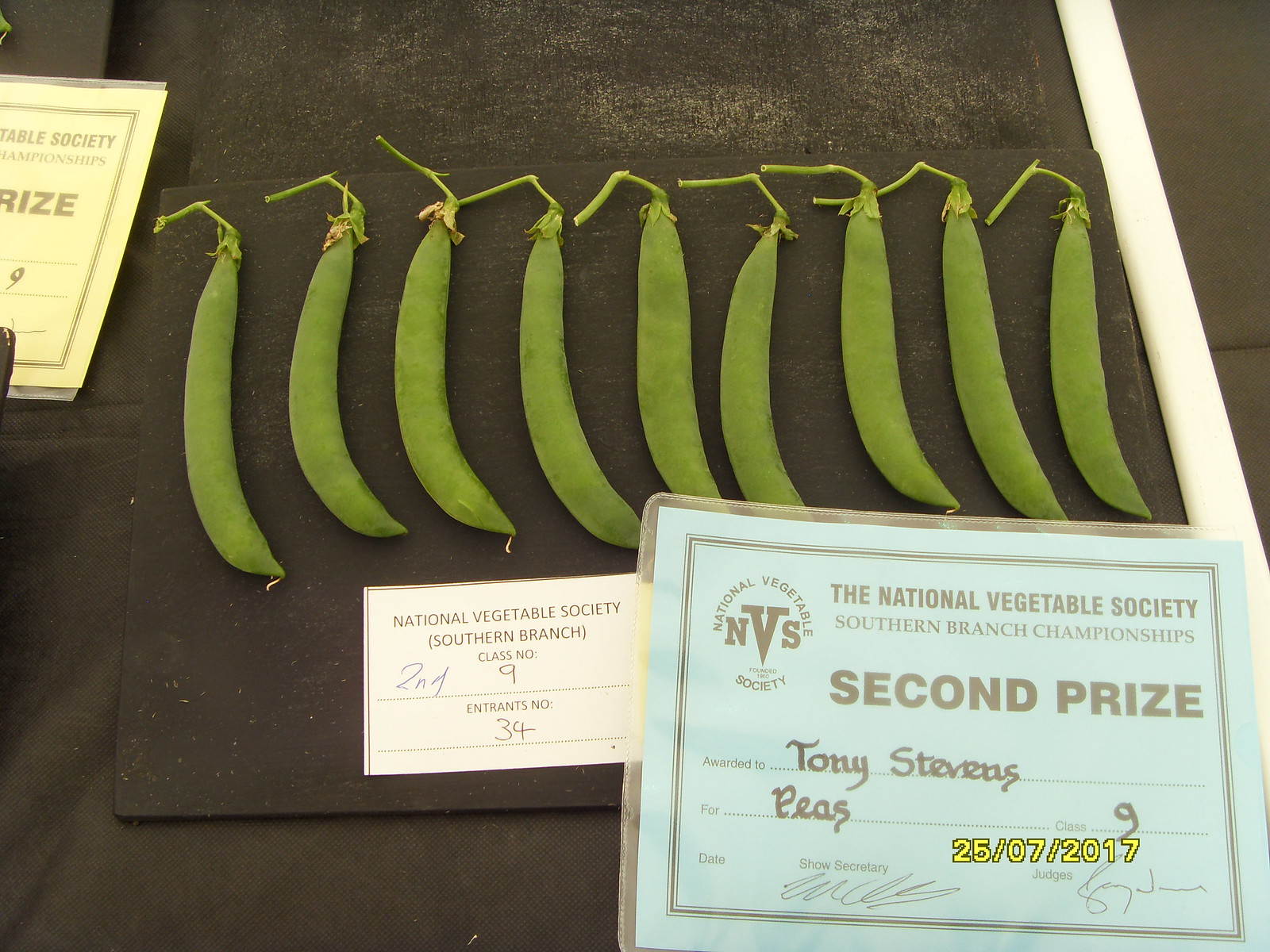This detailed image shows a wooden board serving as a display platform for nine green pea pods, neatly arranged in a row from left to right. In the foreground, prominently featured on the same board, is a white card that reads "National Vegetable Society, Southern Branch," indicating Class No. 9 and Entrance No. 34, signifying its entry into a vegetable competition. A blue laminated certificate is positioned in the bottom right corner of the photo. This certificate is from the National Vegetable Society Southern Branch Championships, awarding a Second Prize to Tony Stevens specifically for peas, dated 25-07-2017. In the upper left corner of the image, another partially visible laminated certificate can be seen, though its text is unreadable, adding to the official nature of the scene. The pea pods and certificates collectively tell the story of a proud moment in a vegetable competition, showcasing the meticulous presentation and recognition of the entrants.